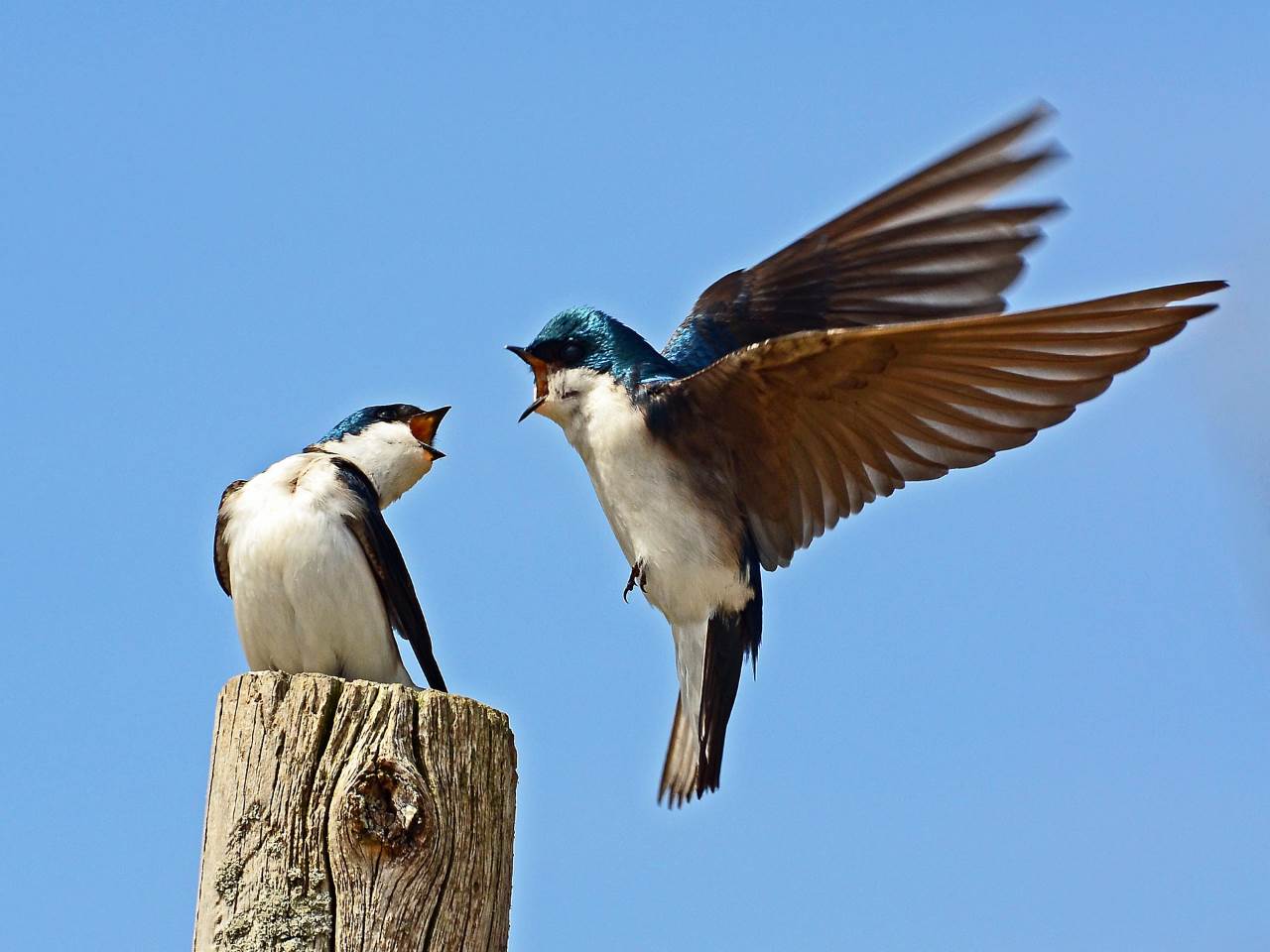The photograph captures a dynamic scene featuring two tree swallows against a clear, pastel-blue sky. One swallow, sporting a white underbelly and a bold blue head, is perched on top of a grayish-brown wooden pole. It appears to be squawking or chirping with its head turned slightly to the right, engaging vigorously with another swallow in mid-flight. This second bird, also with a white front and blue head, has its wings spread wide and mouth open, suggesting they might be in a heated argument or animated communication. The background is a pristine blue sky, devoid of clouds, enhancing the focus on this intense avian interaction.